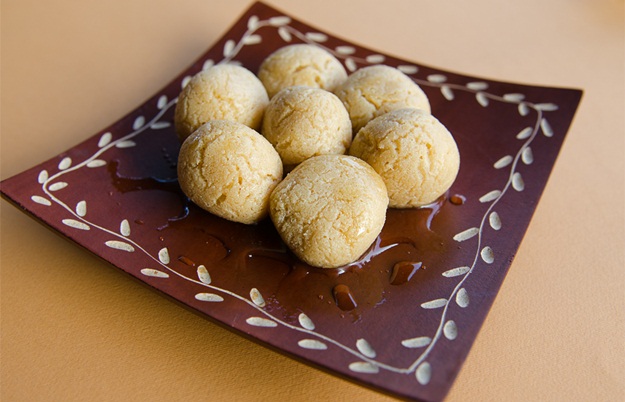This photograph features a square brown plate with ornate white vine and leaf decorations along the border. The plate is presented at a diagonal angle, giving it the appearance of a diamond. Nestled in its slight central indentation are seven round, light brown cookies, possibly snickerdoodles. These cookies exhibit fine cracks on their surface, suggesting they are sweet and slightly squishy. Additional detail includes several drops of what seems to be water on the foreground of the plate. The background of the image is a pale orange, adding a warm contrast to the scene.